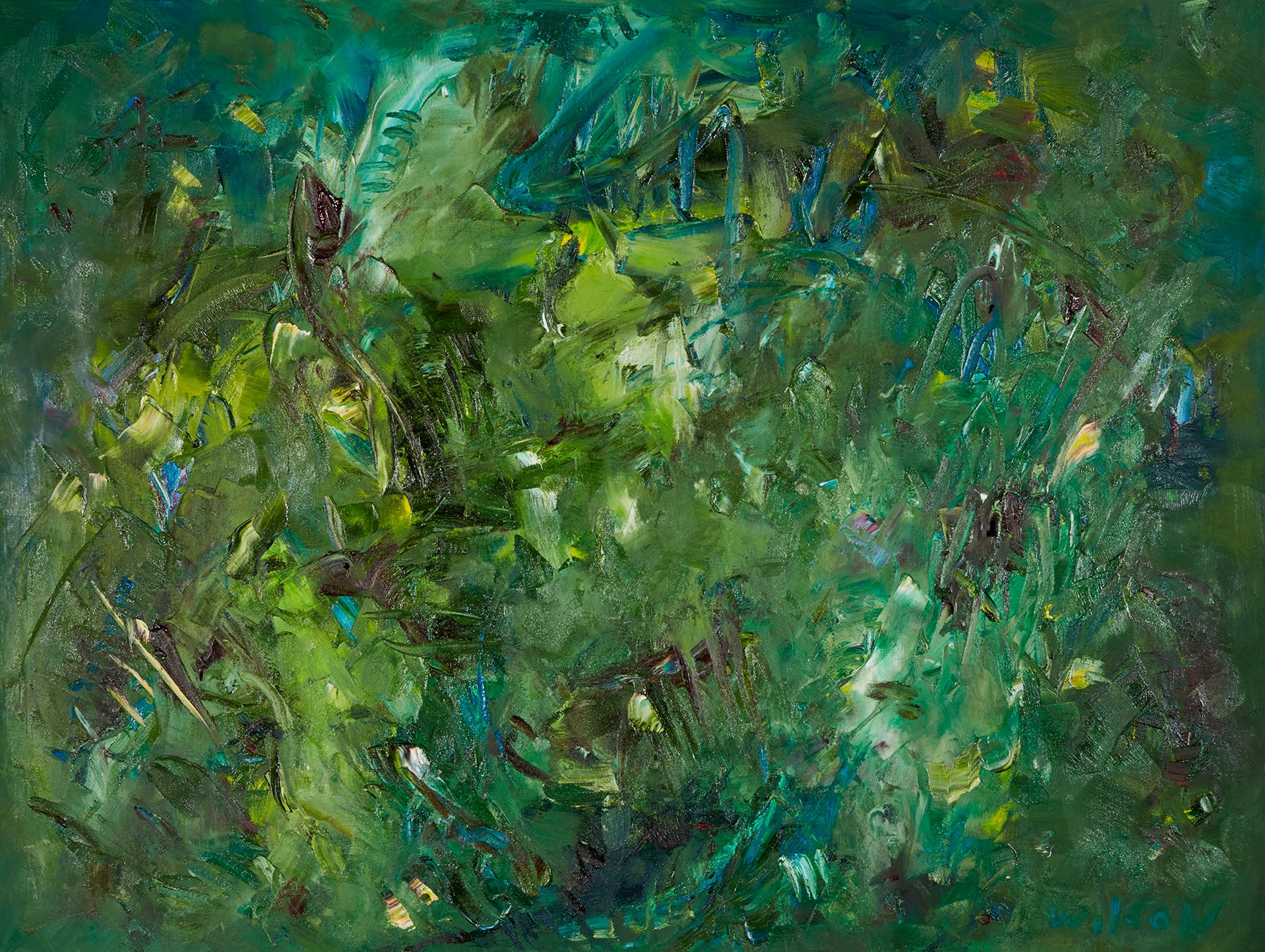This image displays a compelling work of abstract art created with acrylic paints. The artwork, rectangular in shape and measuring approximately six inches wide by five inches tall, features a vibrant assortment of colors applied with various brush techniques, resulting in a richly textured surface. Predominantly, the painting is composed of a dark forest green, which frames the piece along its edges. The central area presents an intricate blend of smudges, swipes, and streaks in assorted shades of green, ranging from bright yellows to minty blue-greens. Interspersed among these greens are streaks of dark brown, almost black, and lighter tones of brown, from tan to mahogany. Off-white or beige splashes of color punctuate the composition, enhancing its complexity. The artist’s application of the paints, with heavy layering and swirling motions, not only creates visual interest but also offers a tactile experience, inviting the viewer to feel the varied textures that characterize this expressive and chaotic arrangement of colors.